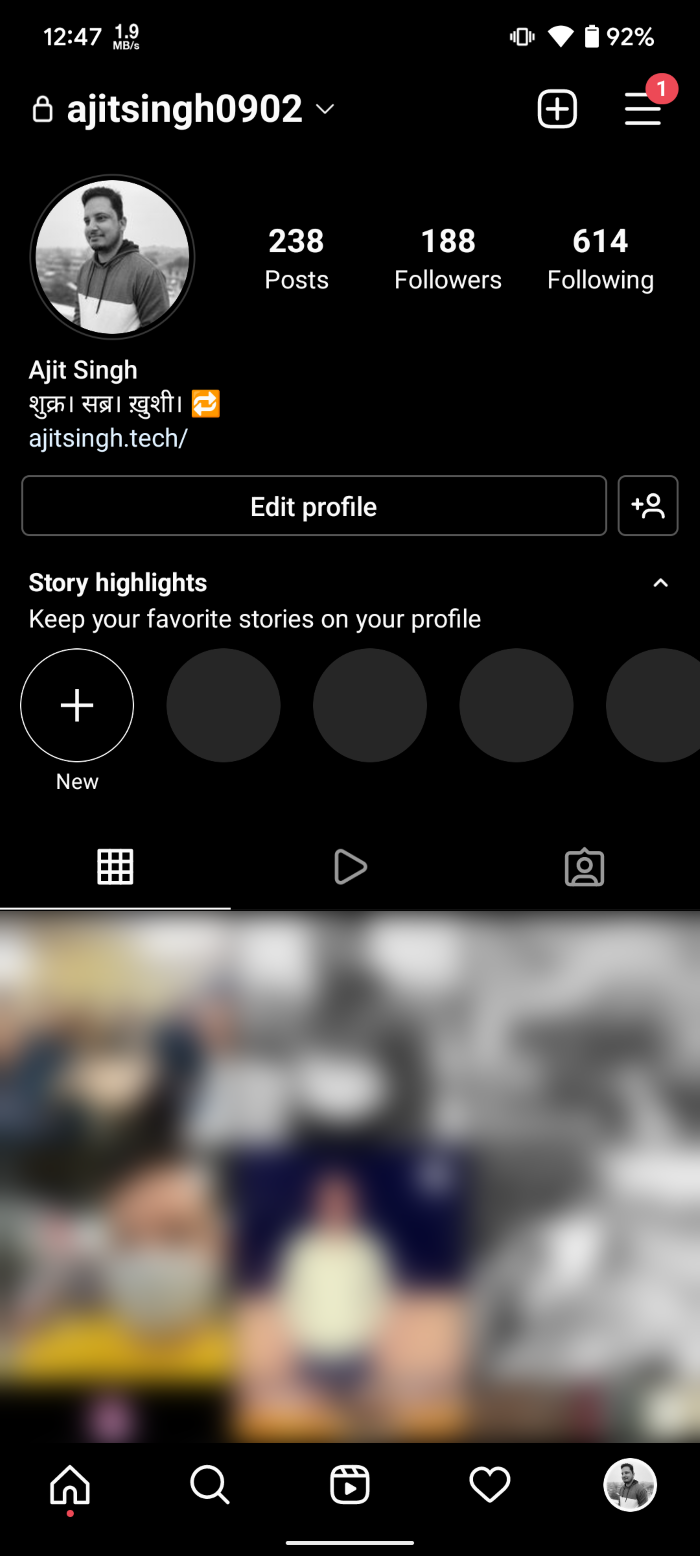The screenshot showcases a social media profile page with the username "A-J-I-T-S-I-N-G-H-0902." Displayed prominently, the profile picture is of a man gazing to the left while outdoors, wearing a hoodie with a white bottom and dark-colored top. The profile details include 238 posts, 188 followers, and he is following 614 people. Additionally, there is an "Edit Profile" button visible below his name and address.